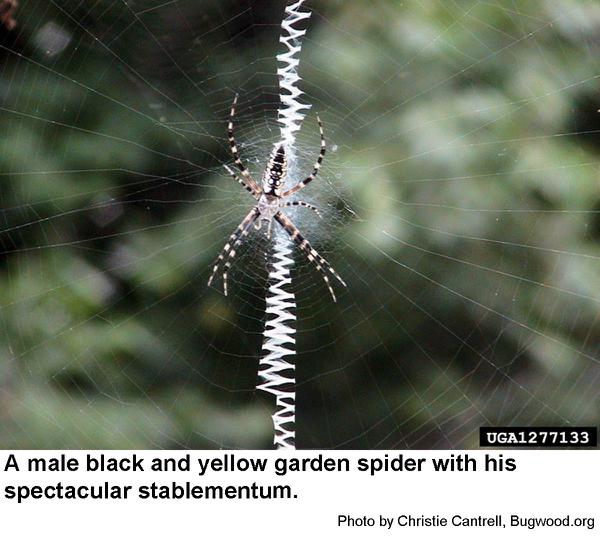The image is a detailed close-up of a large male black and yellow garden spider, prominently positioned at the center of its intricately spun web. The spider exhibits a striking pattern of black, white, and tan stripes extending along its long legs and large body, reminiscent of zebra stripes. The web itself features a prominent and dense zigzag pattern, termed a "spectacular stablementum," running vertically through the middle, composed of thick, closely woven silk. Surrounding this central section, the web expands into finer, thin strands that radiate outward. The background of the photo is a blurred expanse of green foliage, providing a stark contrast to the detailed foreground, yet lacking visible detail. Below the photograph, the text reads "a male black and yellow garden spider with his spectacular stablementum," followed by "photo by Christy Cantrell, bugwood.org." Additionally, there is a black box on the bottom of the image displaying the code "UGA1277133."